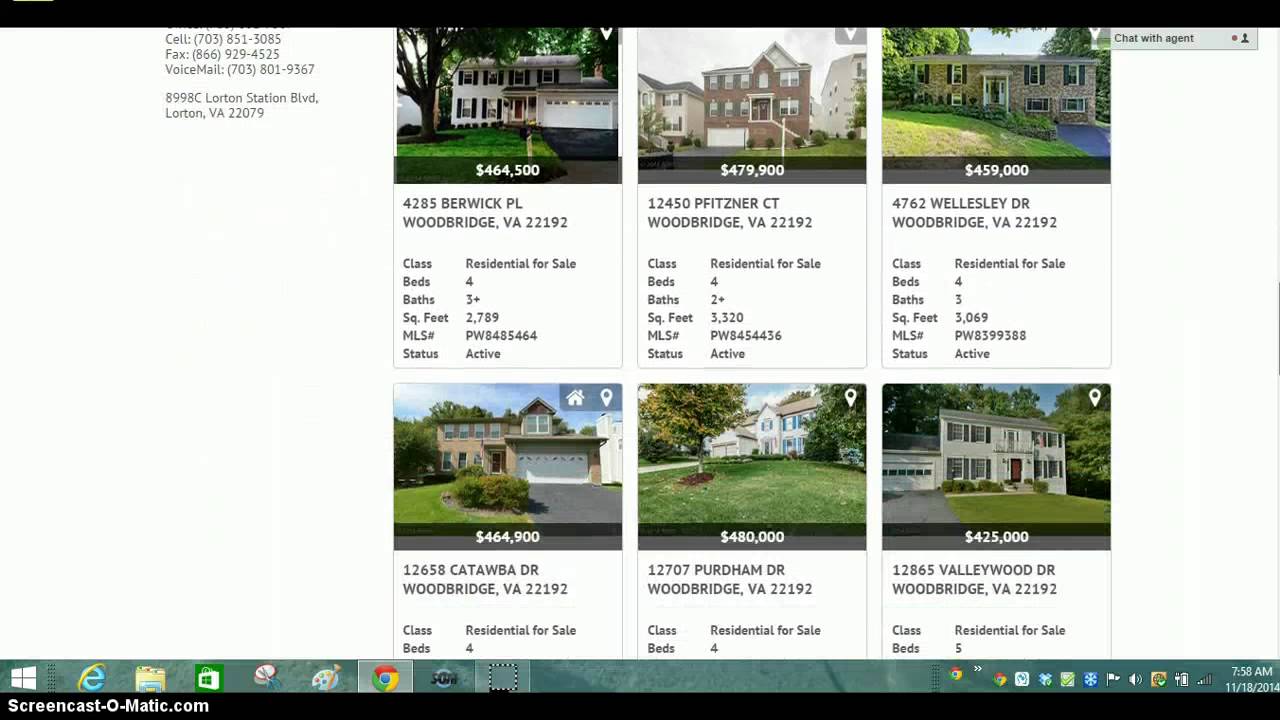Screenshot of a real estate website viewed on a computer screen, featuring six different property listings in Woodbridge, Virginia. Each listing displays a single exterior photo of the house, followed by its price and brief details. The prices range from $425,000 to $479,000. The website's identity is not discernible from this image.